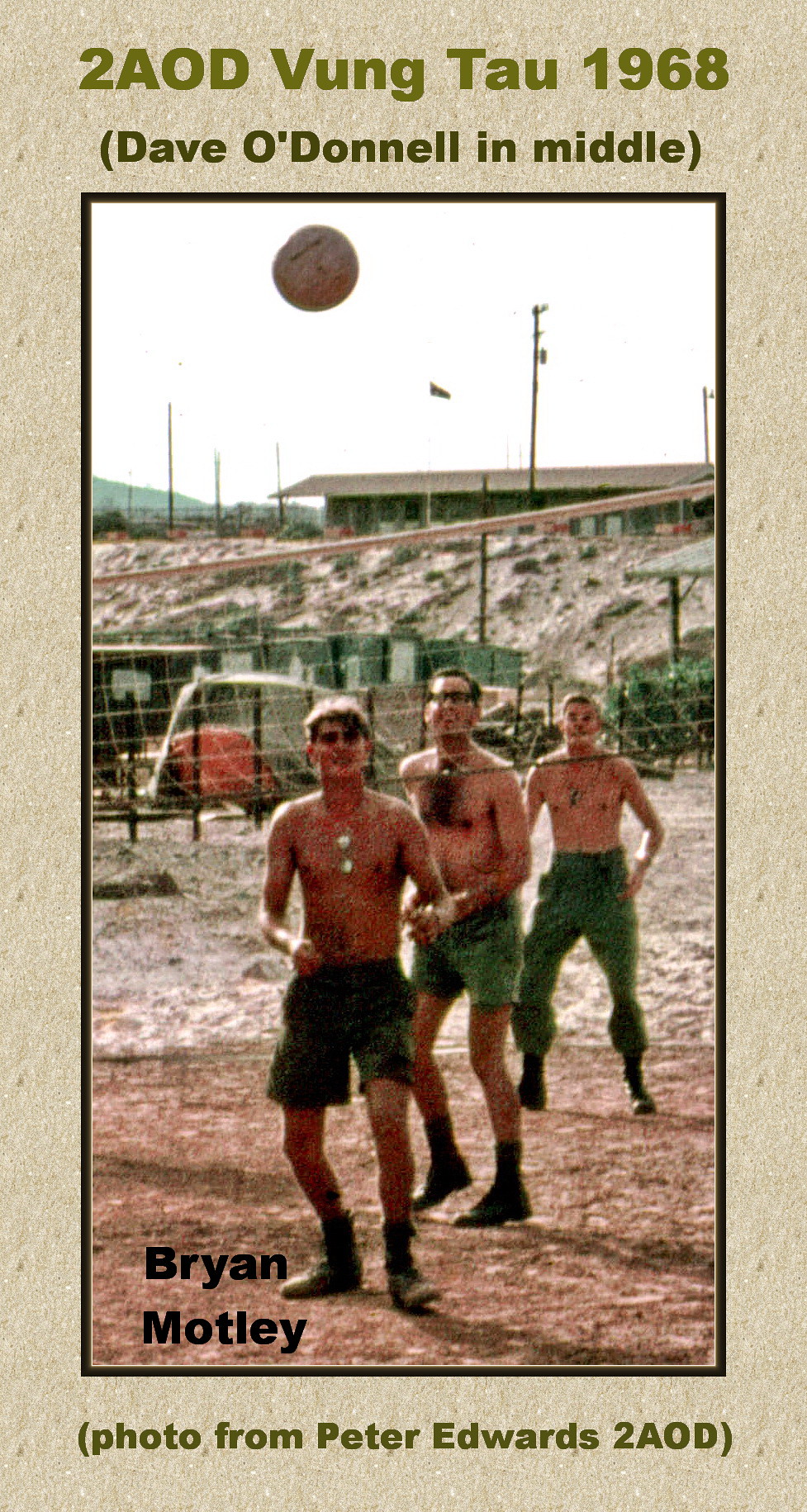In this vintage, grainy, and slightly yellowed photograph, three young shirtless men, presumably soldiers given their dog tags, stand on a brown, rocky, and minimally vegetated terrain, possibly a beach. They are playing a game of volleyball, as evidenced by the net in front of them and the volleyball suspended in the air above their heads. Each man wears green shorts and boots, suggesting a military uniform common during the Vietnam War era. In the background, there are green barracks and power poles under a white sky, indicating an outdoor military facility. The portrait-oriented photo is bordered in brown and features several captions: at the top, "2AOD, Vung Tau 1968" and "Dave O'Donnell in the middle," while the bottom left corner reads "Brian Motley." Additionally, "Photo from Peter Edwards, 2AOD" is noted. This snapshot encapsulates a moment of leisure during a tumultuous period, offering a glimpse into the daily life of soldiers stationed in Vietnam.